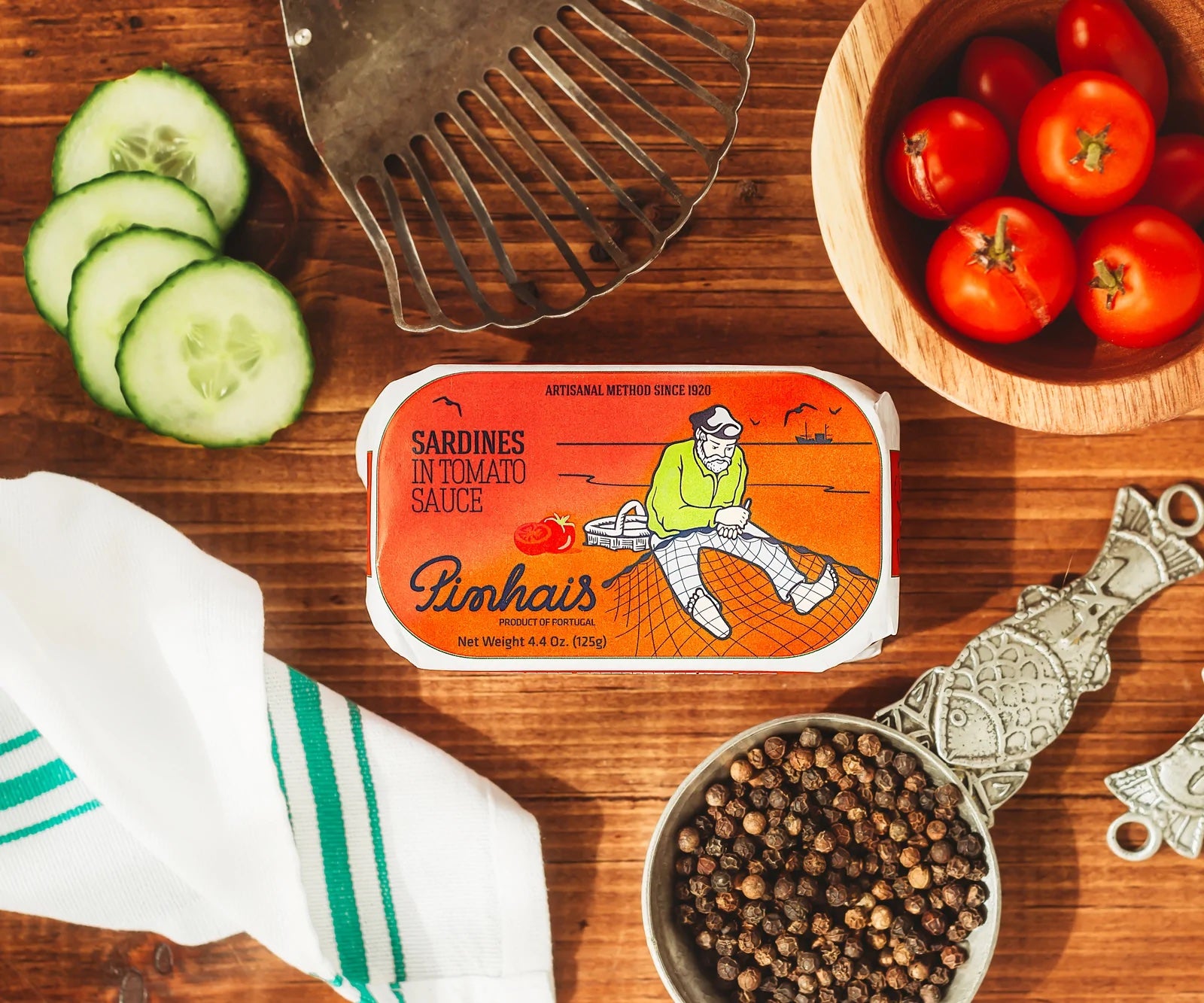This square, full-color photograph is a meticulously staged top-down view of a stained brown wooden table. The wood's grain is easily visible, adding a rustic feel to the image. In the center lies a rectangular sardine can with curved corners, featuring an orange label decorated with a cartoonish illustration of a fisherman working on his net, accompanied by a ship on the horizon and birds in flight. The packaging includes the text “Pinhais Sardines in Tomato Sauce, Product of Portugal, Net Weight 4.4 ounces (125 grams), Artisanal Method Since 1920” in black. 

In the top right corner, a wooden bowl is filled with bright cherry tomatoes, while the top left corner showcases four slices of cucumber and an old, worn-out metallic spatula just below them. A white cloth with green stripes is neatly folded in the bottom left corner, contrasting subtly with another bowl at the bottom right. This unique bowl, crafted to resemble the side of a fish, contains unground black peppercorns. The overall arrangement of these food items and objects, lit by artificial indoor lighting, emphasizes a harmonious blend of textures and colors on the brown wooden surface.